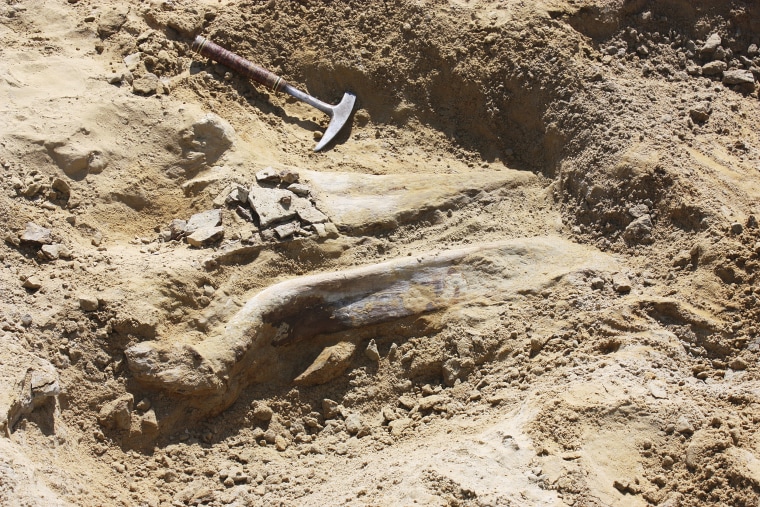The image depicts an excavation site characterized by varying shades of light to dark brown, dry sand, and gravel. Dominating the scene is a small hammer with a dull silver head and a semi-reddish round handle, positioned at the top of the image. Surrounding the hammer are scattered fragments of broken rocks and sediment ranging from light gray to light brown. The landscape appears dry, indicating it hasn't rained in a long time.

Central to the image is an area where active digging has occurred, revealing what seems to be bone structures, potentially from an animal. The exposed bone exhibits white parts protruding from the clay-like soil, with some pieces still partially buried under the sediment, particularly towards the left-hand side. The uneven terrain shows the higher dirt level at the top transitioning to a lower level towards the bottom, highlighting the depth and layers unearthed during the dig. Additionally, remnants of cloth or materials that may have been used during the excavation are visible, adding to the intricacies of the site.